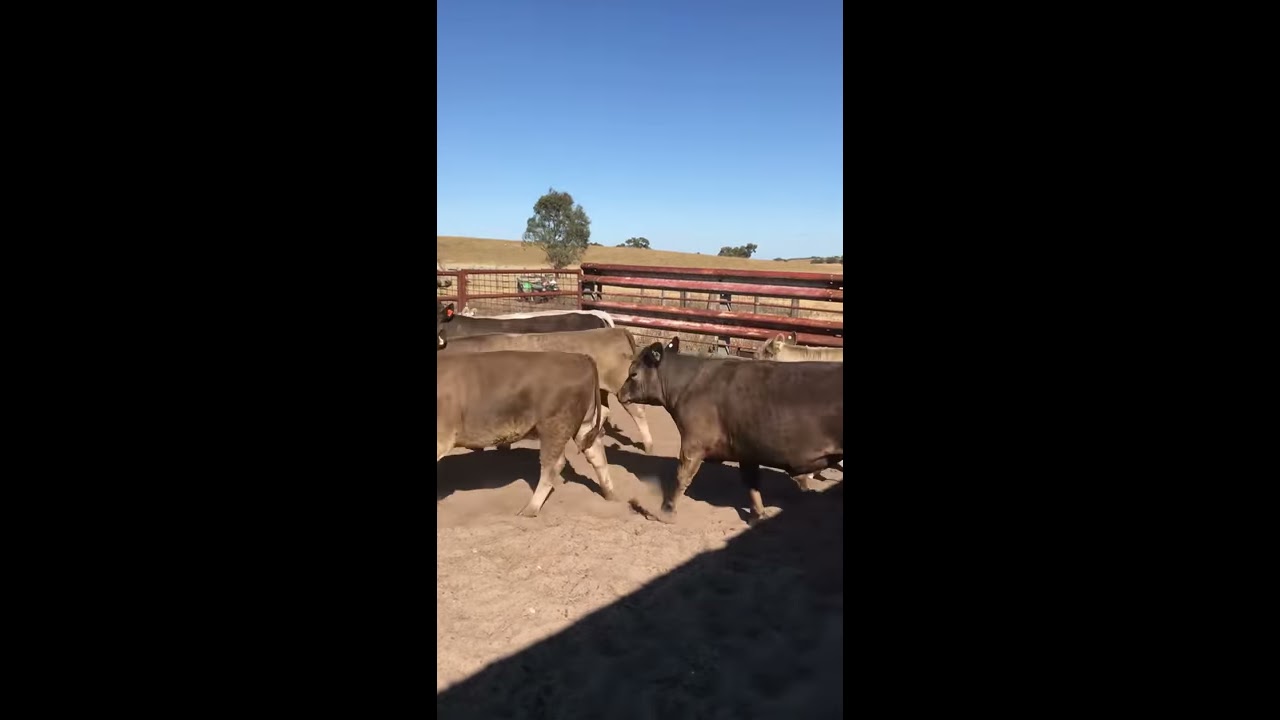This is a detailed, horizontally aligned image showcasing cows in a secluded, enclosed area on a farm. The focal point reveals five cows, primarily brown, with one partially white cow, roaming on sandy dirt within a rustic red fence. Some cows are walking while another, possibly lying down, is partly obstructed. The cows' left ears are visible, featuring orange tags. A clear, bright blue sky extends across the top of the photo, emphasizing the lush, grassy fields and sporadic trees in the distance. A small green tractor can be seen in the background, hinting at ongoing farm work. The sides of the image are solid black, framing the central vertically-shaped picture.